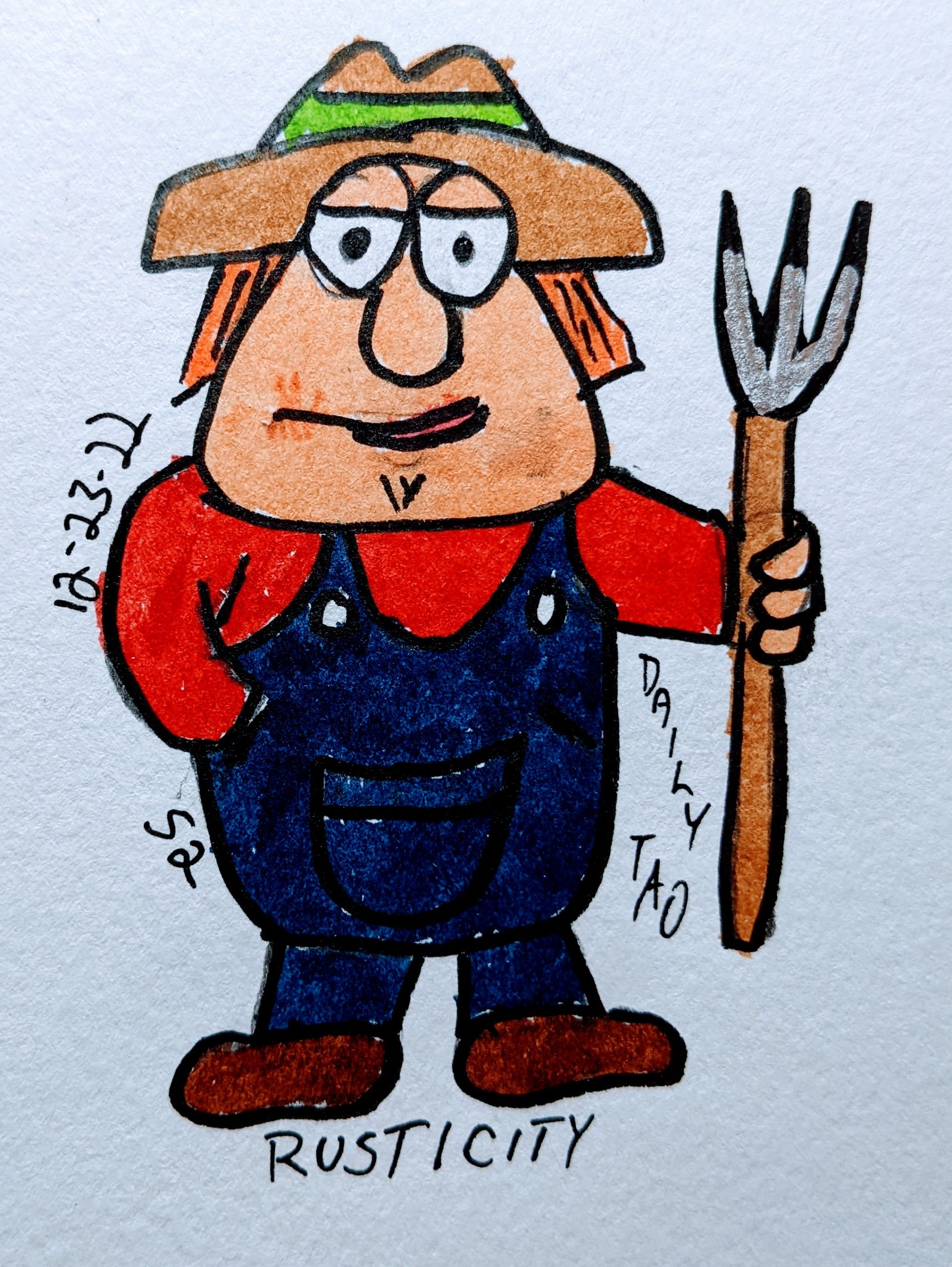The image is a color photograph of a cartoon drawing, created with marker pens, depicting a farmer positioned directly in the center. The farmer has a triangular, A-shaped head with large round eyes, a small round nose, a partially open mouth that suggests a smile, and a hint of a chin. He is wearing a brown hat adorned with a green band, has ginger hair, and is dressed in dark blue overalls over a red shirt. He has brown shoes on and holds a three-pronged pitchfork in his left hand while his right hand is tucked into his overall pocket. The background is a bluish-gray, and the drawing is on white paper or card. Surrounding the farmer, there is black handwritten text: "12-23-22, S2" appears on the left, "Daily Tao" is on the right, and "Rusticity" is written at the bottom under the farmer’s boots. The image captures the essence of a child's drawing with simple dimensions, light lime green, light brown, darker browns, grays, blacks, dark blue, red, and darker brown colors. The rustic city setting adds to the charming simplicity and warmth of the illustration.